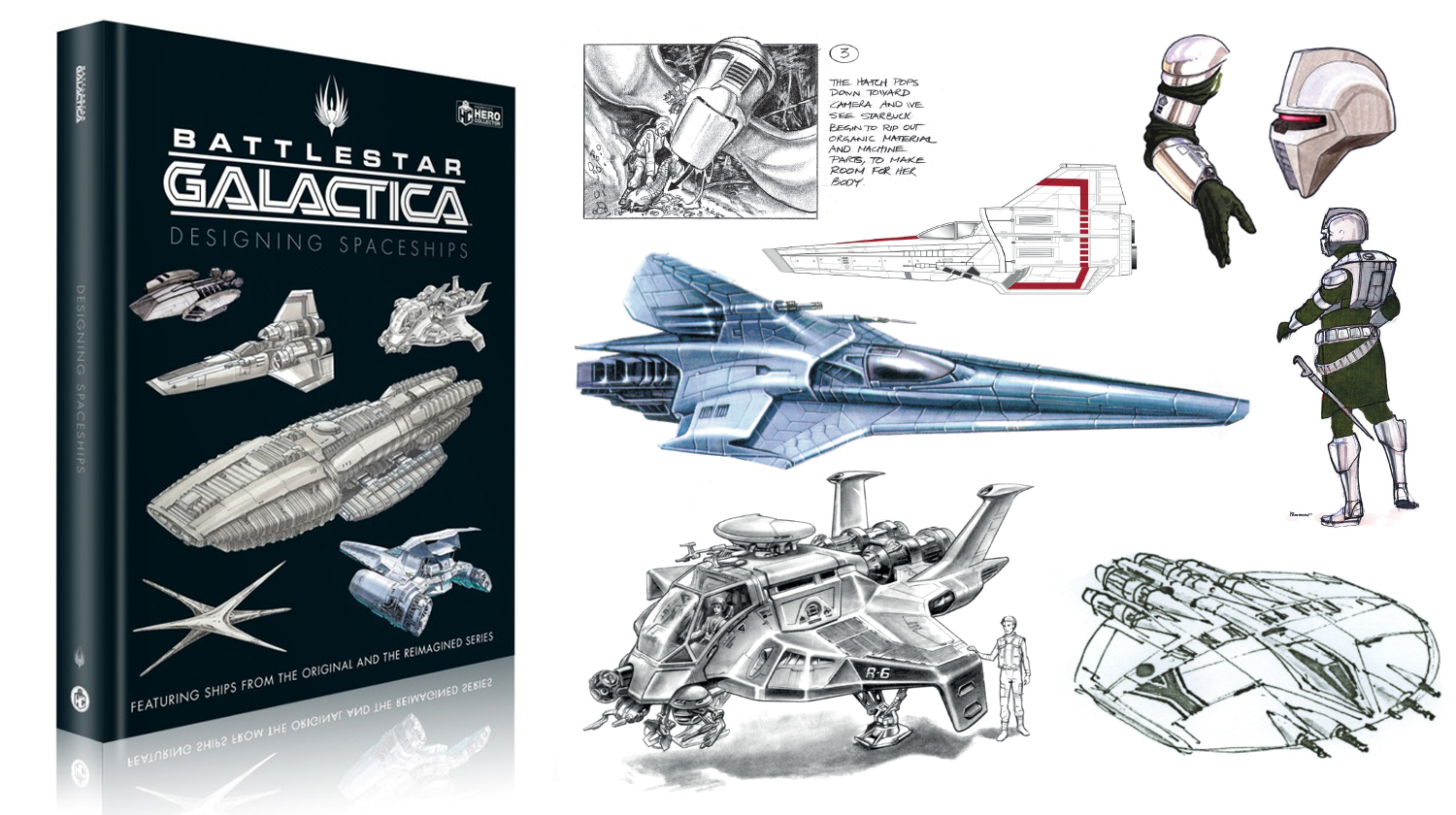The image features an open book titled "Battlestar Galactica: Designing Spaceships," positioned against a white background with a faint gradient and a subtle reflection below the book. The hardcover book has a black cover with large, futuristic white text at the top reading "Battlestar Galactica," and smaller text underneath that says "Designing Spaceships." The cover showcases six black-and-white illustrations of various spaceships from the series. At the bottom of the cover, thin white text states, "Featuring ships from the original and the reimagined series."

To the right of the book cover, a prominent interior page from the book is displayed, highlighting concept designs of well-known ships and characters from the original Battlestar Galactica series. Featured illustrations include detailed drawings of several spaceships, such as a shuttle with a white exterior and red accents, another ship with a design reminiscent of a flying saucer, and one with a helicopter-like appearance. Additionally, the page includes designs of the Cylons, the primary antagonists of the show, showcasing their silver helmets and black and silver armor. The detailed artwork demonstrates the intricate concept designs that bring the sci-fi universe of Battlestar Galactica to life.